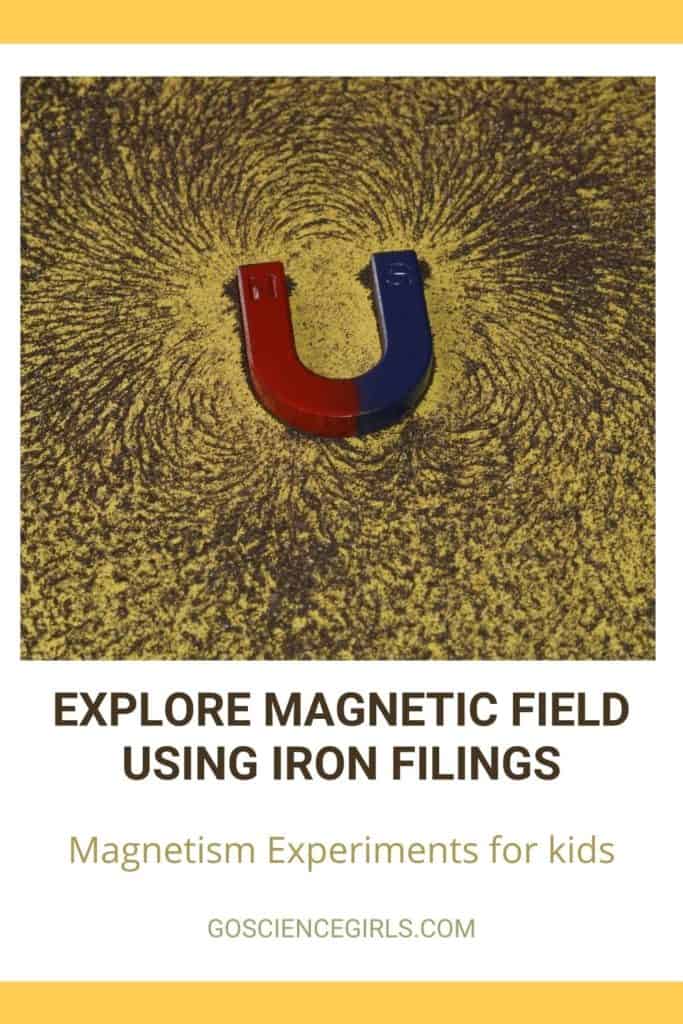The image featured in this informational post highlights a magnetic experiment designed for kids to explore the concept of magnetic fields using iron fillings. At the center of the image is a prominent horseshoe-shaped magnet, vividly colored with the left half in red and the right half in blue. Surrounding the magnet, iron fillings create intricate and beautiful magnetic lines, vividly illustrating the magnet’s influence. The magnet rests on a yellow surface, giving a clear contrast to the black iron fillings that resemble fine hairs scattered around it. The top and bottom sections of the image are framed by solid medium yellow-orange banners. Below the magnet, black text reads: "Explore Magnetic Field Using Iron Fillings. Magnetism Experiments for Kids. GoScienceGirls.com," directing viewers to the educational website. The overall composition of the image, with its vibrant color contrasts and clear demonstration of magnetic fields, offers a visually captivating and informative experience.